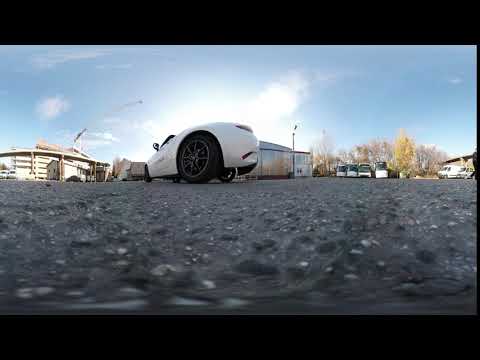The image captures a panoramic view of a private parking lot taken from a low angle, almost at ground level, highlighting the dark gray, grainy asphalt interspersed with numerous tiny white rocks. At the center of the image stands a white two-door coupe, prominently viewed from the side to the back, featuring black rims and tires. Beyond the vehicle, the background showcases two distinct buildings: on the left, a white building with several pioneers stationed in front, and directly behind the coupe, a modern structure with multiple glass walls. To the right of this glass building is a row of four white vans parked in alignment. The scene is set on a cloudy, yet bright day, indicated by the diffused sunlight filtering through, suggesting it's either midday or early afternoon. The backdrop hints at a fall setting with sparse trees visible behind the vehicles.